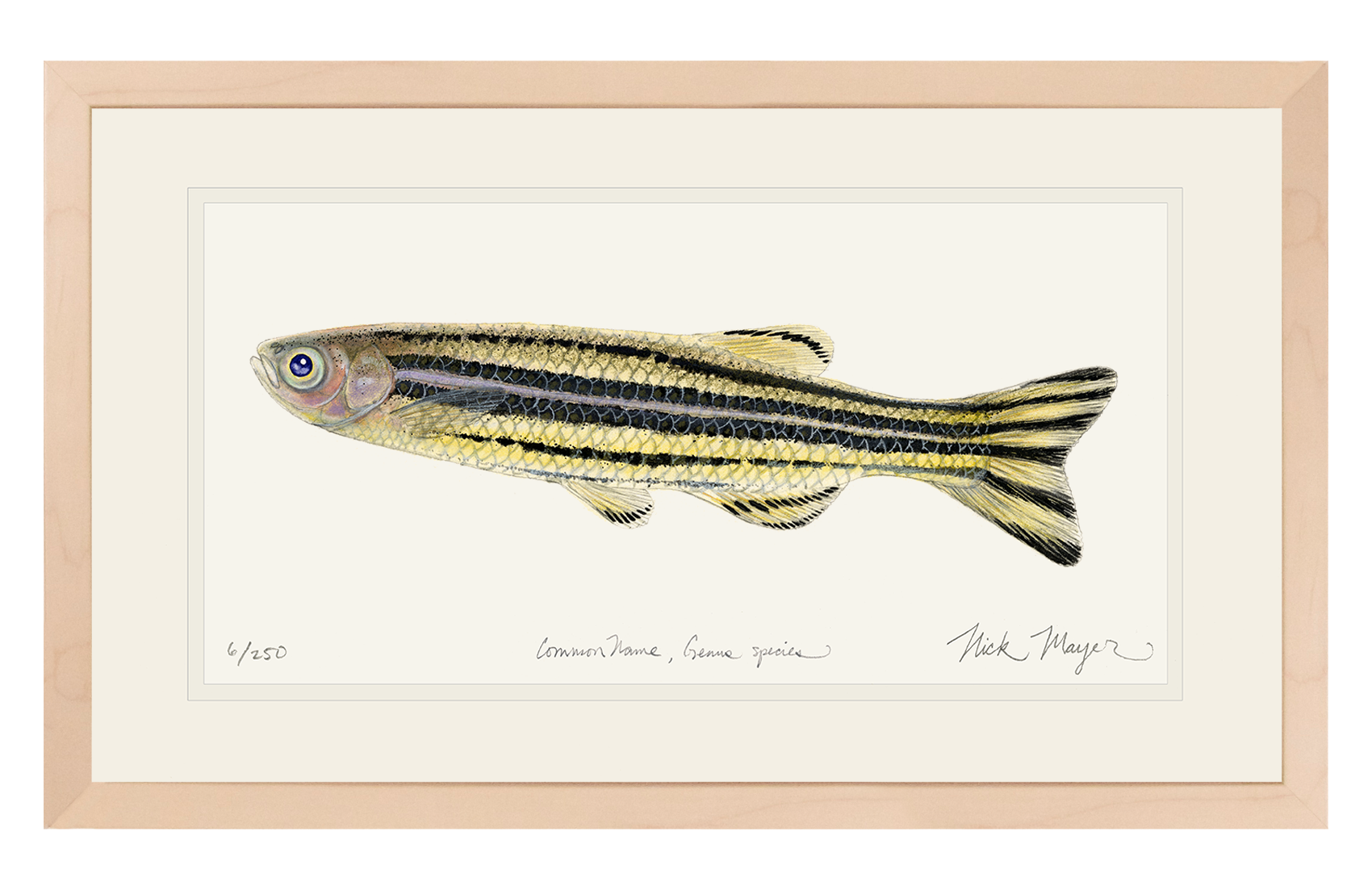This striking image, possibly a lithograph or painting, showcases a yellow-scaled fish adorned with horizontal black stripes that run from just behind the head to the tail fin. These distinctive stripes are complemented by a single silver line along the midsection. The fish's head features a slight tinge of pink and faint brown hues, enhancing its realistic essence. The eye exhibits a reflected light, giving it a lifelike look, while its bottom jaw appears to be pointing upwards, perhaps suggesting it is looking upwards as well.

The fish's fins, including the tail fin and the prominent top fin, are decorated with a combination of yellow and black stripes, with the top fin highlighted by visible rays and a black curved line at the top outline. Additionally, the body is covered in shimmering gold scales that extend from the head to the tail.

The artwork is framed with a lighter white-creamy inner border followed by a light brown outer frame, providing an elegant contrast to the white background of the fish illustration. In the lower left corner, it is marked as "6/250," indicating it is part of a limited edition print run. The lower center area of the image includes the common name and scientific classification of the fish, while the bottom right bears the signature of the artist, Nick Mayer. 

Overall, this beautiful and detailed fish image, with its impeccable coloration and border detailing, is a testament to fine artistic craftsmanship.